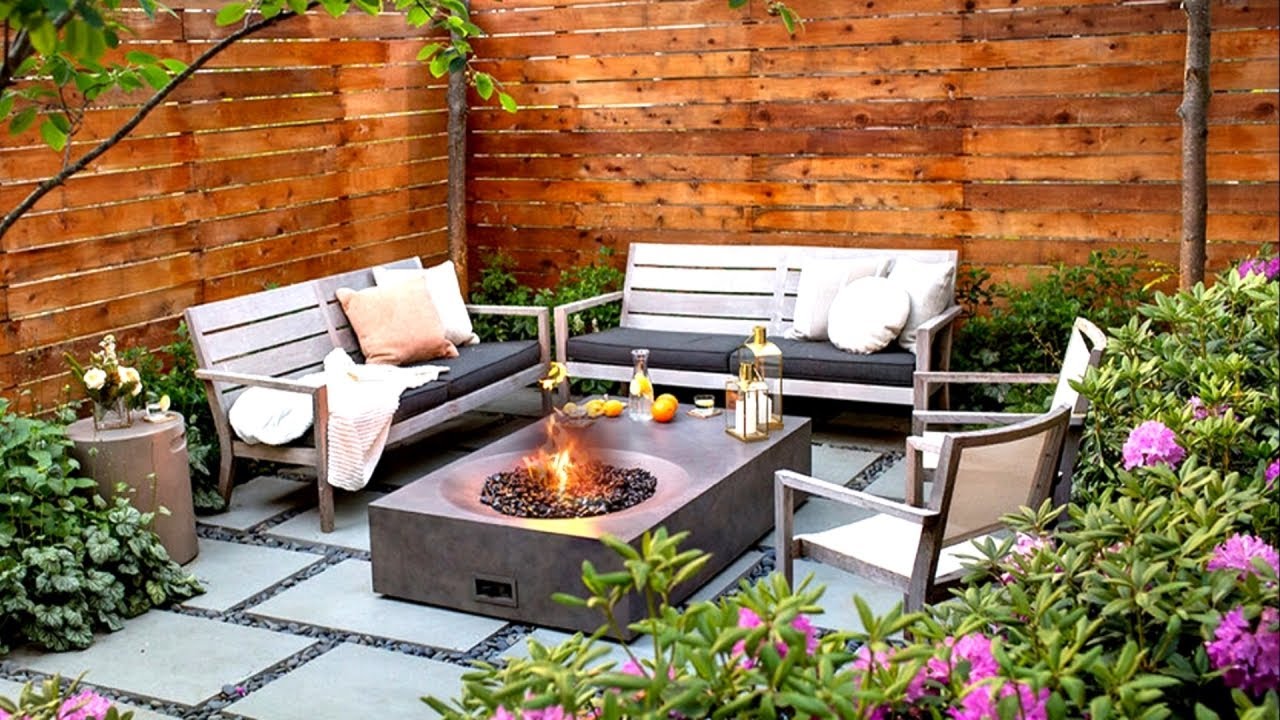Set in a private backyard, the image captures an inviting outdoor space enclosed by a weathered brown wooden fence that ensures seclusion. Central to the setting is a steel gray gas fire pit with a vivid red and yellow flame dancing over black stones. Flanking the fire pit are two comfortable gray couches, each seating two people, adorned with a mix of dark gray square cushions, a circular cushion, and a blanket draped over the left couch. Two matching chairs complete the seating arrangement.

The ground is a thoughtfully designed patio featuring large pavers interspersed with granite chips, echoing the charm of a brick house. On the table beside the couches, there's a decanter and a carafe containing a citrus-infused drink, accompanied by two oranges and several lemons. Two brass lanterns sit adjacent, adding a warm glow alongside candles protected in glass holders. 

The space is enhanced by lush greenery, including rhododendrons in bloom with green and lavender hues on the right-hand side, small bushes lining the fence, and two trees—one slightly left of center and another to the far right. Notably, a decorative sculpture of an elephant with a rider adds an artistic touch to the area, blending seamlessly with the tranquil yet rustic atmosphere of this cozy outdoor retreat.